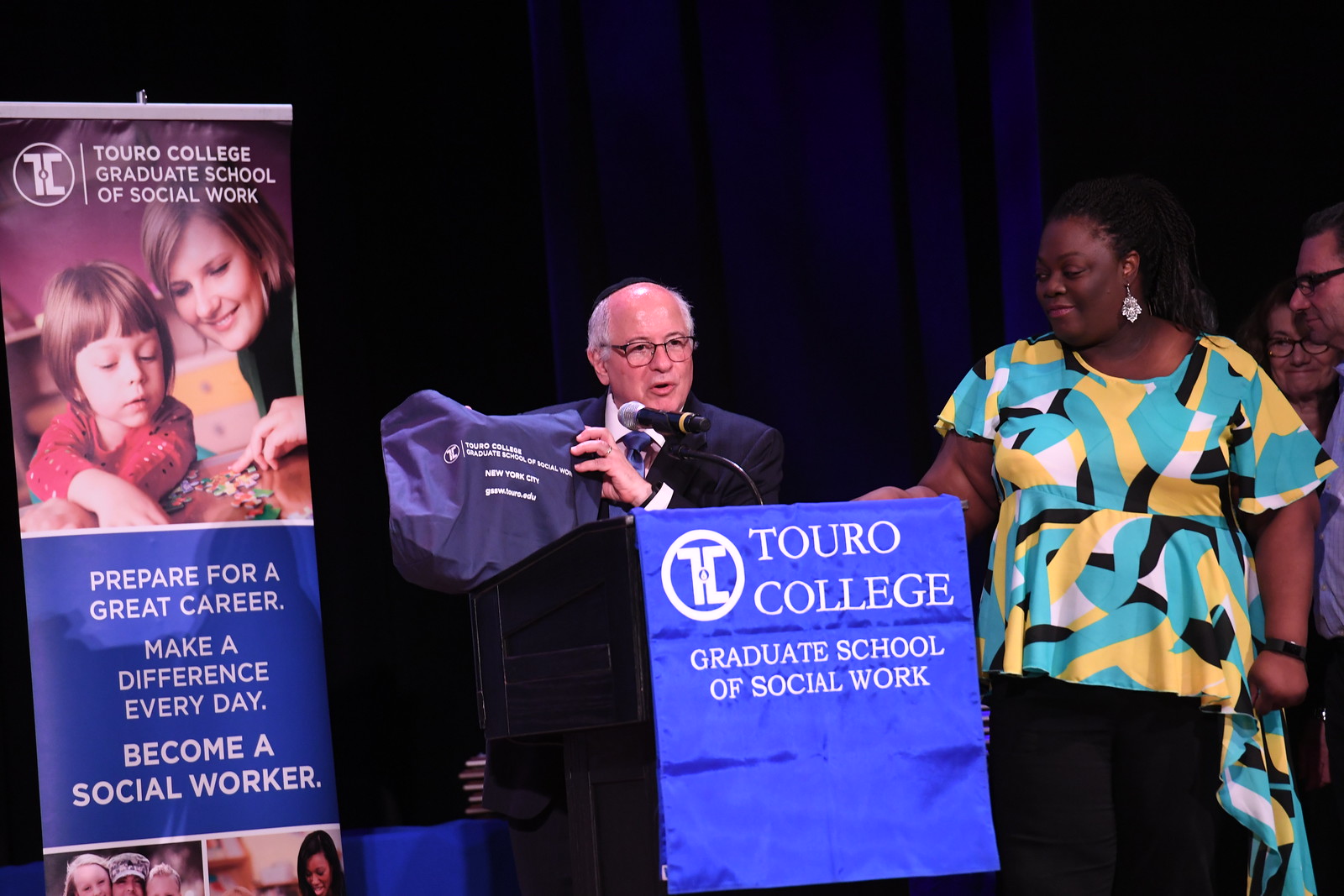In this photograph, a group of individuals is positioned on a stage, likely during a graduation ceremony. At the forefront, a distinguished older white male with white hair and eyeglasses stands at a black podium, speaking into a microphone. He is dressed in a black suit and is holding up a blue piece of fabric, which could be a t-shirt or a canvas bag. The fabric bears the inscription "Touro College, Graduate School of Social Work, New York City" in white print alongside the college's logo.

Prominently displayed on the front of the podium is a blue banner that also reads "Touro College Graduate School of Social Work." Directly behind the gentleman is a tall sign featuring various images of women and children and additional text in white on a blue background that reads, "Prepare for a Great Career, Make a Difference Every Day, Become a Social Worker."

Standing next to the speaker on his right is a smiling black woman dressed in a vibrant yellow, blue, white, and black blouse paired with black pants. Closer to her is another man, a white male in black glasses, wearing a blue shirt and dark black pants. Behind both of these individuals is a white female with a warm smile and eyeglasses, further adding to the congenial atmosphere of the event.